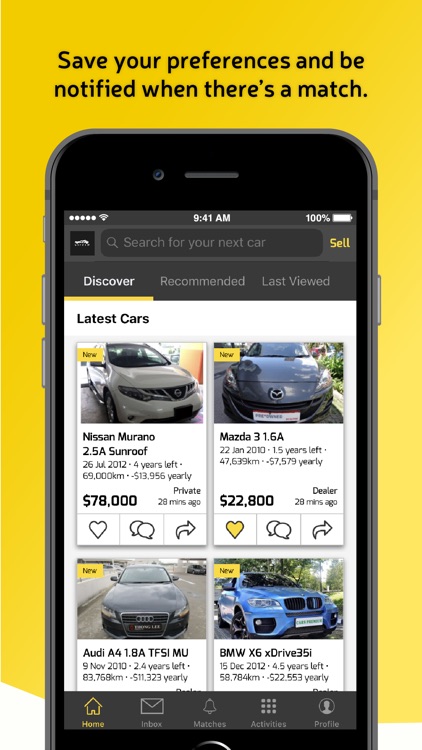A vertical portrait-style screenshot showcases an advertisement or instructional image with a vibrant yellow background. At the top, in bold black font, it reads: "Save your preferences and be notified when there's a match." Below this text, the focal point is a smartphone displaying a page where users can browse various cars for sale. Featured vehicles include a Nissan Murano 2.5A with a sunroof priced at $78,000, a Mazda 3 1.6A priced at $22,800, an Audi A4 1.8A TFSI MU, and a BMW X6 xDrive 35i. However, due to the scroll position, the prices of the last two vehicles are obscured.

The interface highlights a "Discover" button at the top, flanked by "Recommended" and "Last Viewed" tabs. Just above this, there's a search box with a prompt saying "Search for your next car" and a "Sell" button positioned to its right. The status bar of the phone indicates full Wi-Fi signal, the time as 9:41 AM, and a 100% battery level. At the bottom of the screen, navigation buttons are visible for Home, Inbox, Matches, Activities, and Profile. The overall image clearly illustrates a user-friendly search engine for discovering deals on motor vehicles.